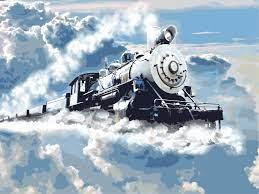This vibrant, color drawing captures a majestic, old-fashioned steam locomotive, depicted in silver and black hues, seemingly traveling through the sky. The train, positioned prominently in the center, powers forward towards the left, its large, round steel front gleaming. Billowing white steam trails from the engine, creating an impression of motion as it plows through a dreamy landscape of blue and white clouds. The perspective offers a slightly upward, left-side view, adding a sense of grandeur and height. Behind the engine, six cars fade into the distance, their diminutive size accentuating the length of the train. The sky above is adorned with shades of blue, with a small patch of blue sky visible in the upper right corner. Despite a fantastical setting, where clouds substitute for tracks beneath the wheels, the crisp detailing of the locomotive and the tranquility of the surrounding sky combine to form an intriguingly beautiful piece.